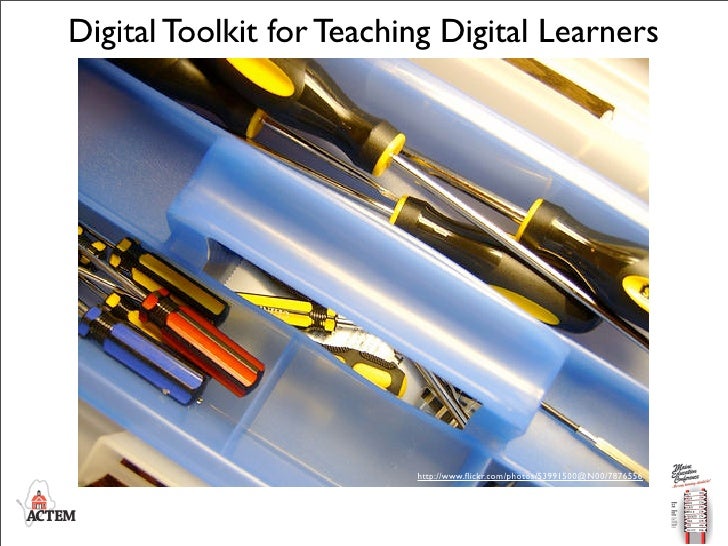The image is a detailed visualization of a toolkit labeled "Digital Toolkit for Teaching Digital Learners" in prominent black text across the top. Beneath the text is a light blue plastic tool container designed with compartments to organize various tools. On the left side, the tray holds screwdrivers with distinctive handles: some are blue and black, others are yellow and black, and there are also red and black ones. Towards the top right of the container, larger screwdrivers have black handles accented with yellow designs, showing the shiny metal tips. The container features a raised handle in the center for easy carrying. In the lower left-hand corner, the letters A-C-T-E-M are displayed in black, next to a small logo with a red bar. On the right side of the image, there appears to be a direction signpost with unreadable black and red text. The overall image looks slightly grainy, possibly indicating it was taken from a textbook or a similar printed material.